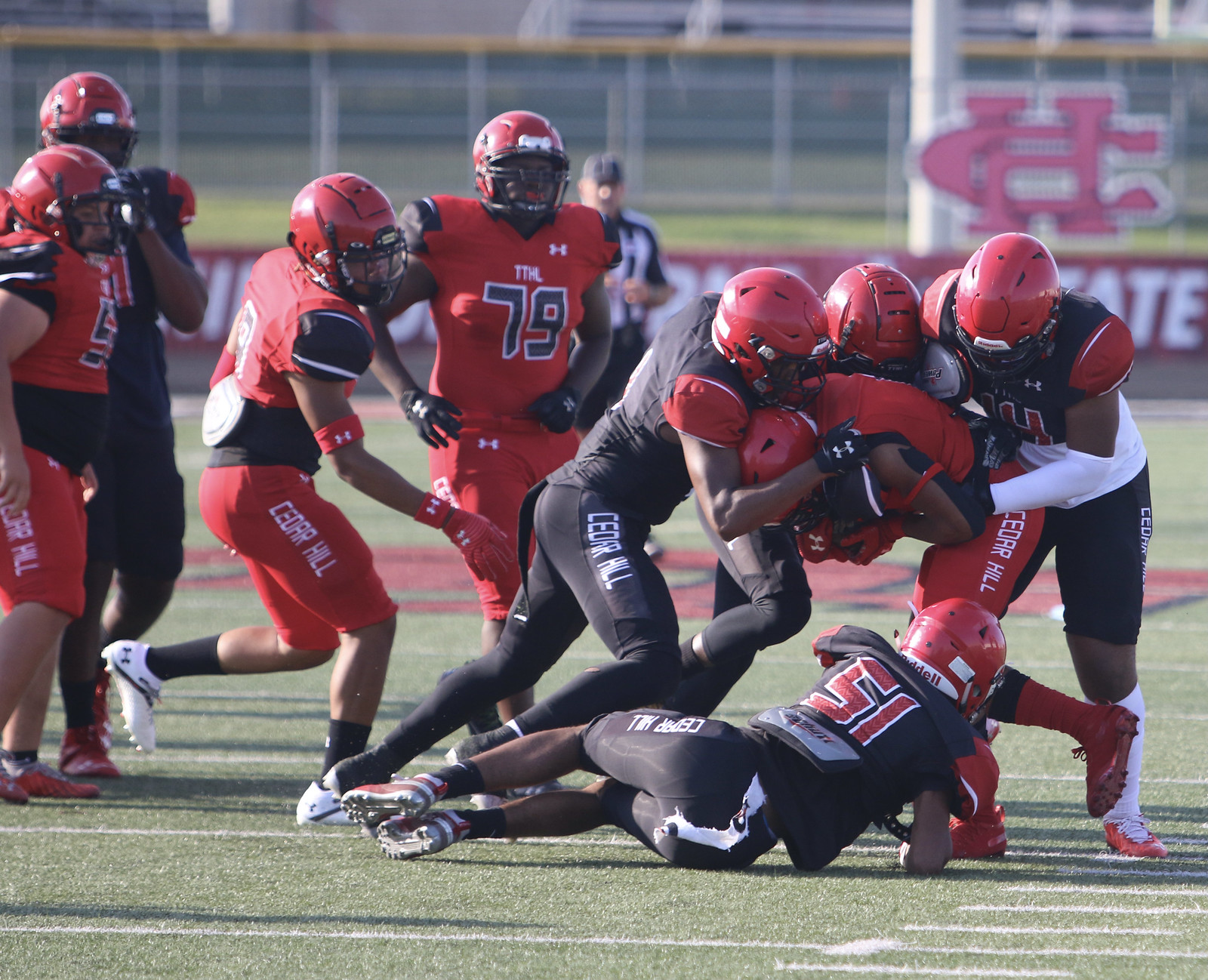This image captures an intense moment during a high school football game at Cedar Hill State stadium. The field is clearly marked with yard lines and hash marks, indicating it’s a regulation football field. In the foreground, several players are prominently featured in action. On the right side of the image, three players in black uniforms with red helmets are tackling a player in a red uniform and red helmet, who appears to be holding the ball. Among them, player number 51 in a black uniform is lying on the ground, possibly grabbing the leg of the tackled player. Nearby, four more players are visible: one in a black uniform, another in a red and black uniform, and two more in red uniforms, including player number 79 and player number 5, whose number is partly obscured. The background includes the stadium with the letters 'C' and 'H' superimposed and the word 'State' visible, affirming this is a Cedar Hill State game. The teams are wearing predominantly Under Armour gear, suggesting they might come from the same school but represent different squads, like offense and defense. The scene is captured in the late evening, evidenced by the long shadows cast on the field.